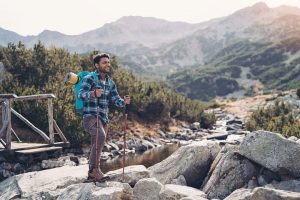In this small outdoor photograph, a man with short dark brown hair, a beard, and mustache is holding two hiking sticks while standing on boulders. He is wearing a blue and white plaid flannel shirt, dark grey pants, dark-colored hiking boots, and a turquoise backpack. The man is looking up and off to the upper right-hand side of the scene with a slight smile. The backdrop features a high, mountainous landscape with stripes of white snow scattered across the peaks, indicating a higher elevation. Behind him is a metal bridge-like structure and a mix of greenery and shrubbery, suggesting a rugged, semi-dry terrain. The clear sky adds to the expansive, open feel of the location, enhancing the sense of adventure in this scenic hiking area.